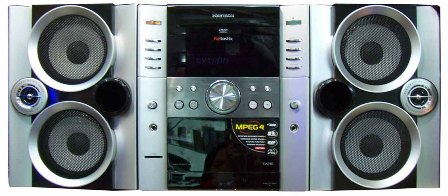This detailed photograph focuses on an old-school stereo system, resembling a vintage boombox. The system features a central silver console flanked by two symmetrical speaker boxes. Both the left and right speaker boxes house two larger speakers on the lower half and two smaller speakers on the upper half, enclosed by a translucent black cover, revealing an intricate multi-layered design with white and black circles.

In the center console, the main control area is also a metallic silver, prominently displaying a large, round volume knob in the middle. Above and below the volume knob are sets of smaller operational buttons; two smaller buttons are positioned on the top, while two slightly larger buttons align at the bottom. Furthermore, each speaker box on the sides is equipped with additional dials, with the left speaker featuring a dial on its left side and the right speaker on its right side.

A distinguishing blue outline highlights one of the larger speakers, adding a hint of color contrast against the otherwise monochromatic silver and black theme of the stereo system. Notably, in the lower right corner of the central console, a yellow sticker reads "MPEG-4". Also faintly visible at the bottom of the console is the reflection of an individual, adding an element of human presence to the image.